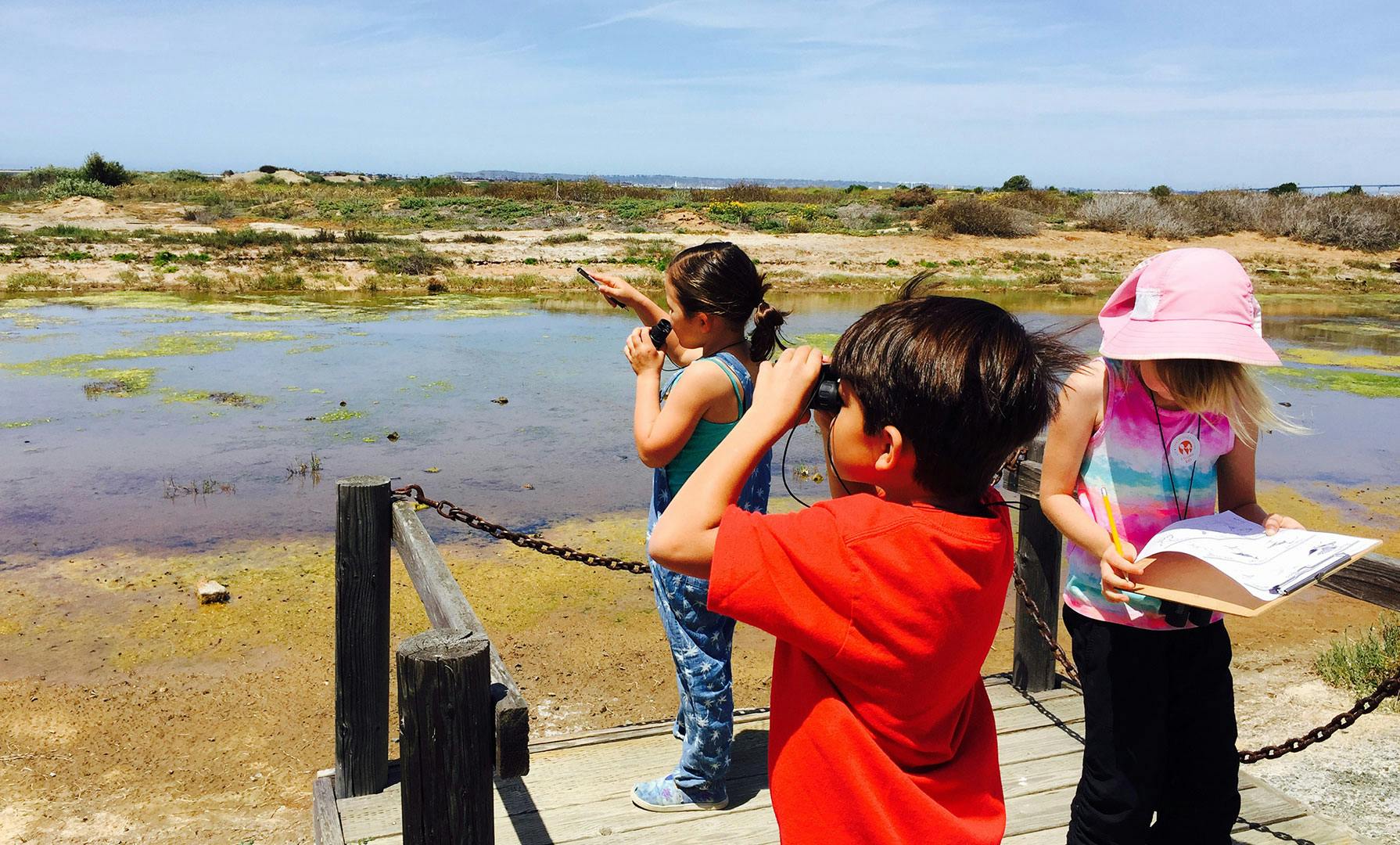In this detailed color photograph, three young children are standing on a wooden dock that appears to be set over a marshland or near a tidal pool area. The dock is bordered by black posts and chains, presumably for safety. The children are gathered in the bottom right quadrant of the image.

The closest child, a little boy with short black hair, is wearing a bright red t-shirt and is holding a pair of child-sized binoculars up to his eyes, gazing out over the landscape. Behind him, a girl dressed entirely in blue—a tank top and blue pants, with black hair—points at something out on the horizon, also using a pair of binoculars. The third child, a girl facing the camera but looking down, is wearing a pink cap and a tie-dye shirt. She holds a clipboard with a piece of paper and a pencil, appearing busy with some sort of worksheet or observational notes.

The surrounding environment consists of a sandy stretch leading into marshland with a small hill and scattered low-growing shrubbery in the distance. The sky is overcast, casting a gray tone over the scene, and the visible water has a grayish hue with tinges of green on its surface. The overall impression is that the children might be on a school field trip or a family outing, exploring the natural landscape.